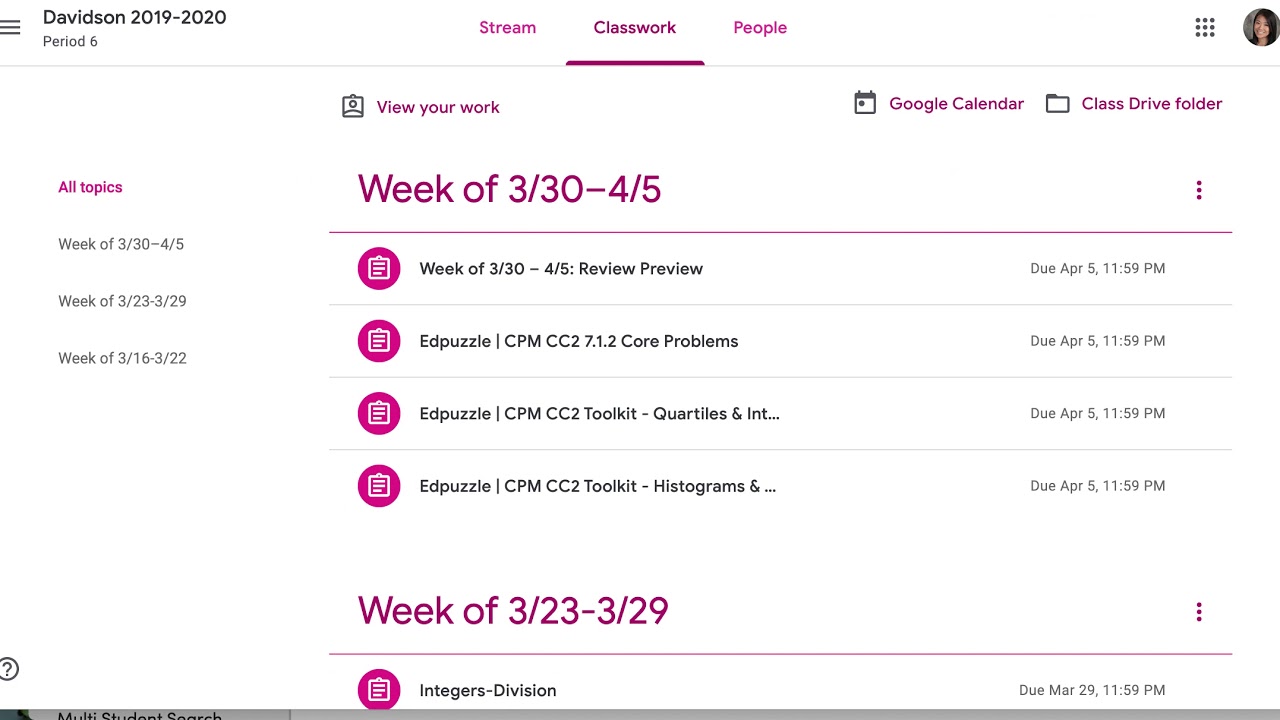This image appears to be a screenshot from an online classroom platform for Davidson High School during the 2019 to 2020 school year, specifically labeled for Period Six. The header section features a white background with text in a fuchsia-pinkish purple color, displaying menu options such as "Stream," "Classwork," and "People." 

On the right side of the image, there's a profile picture of a woman with long black hair, possibly of Asian descent, smiling directly at the camera. Under the "Classwork" section, there's a highlighted purple line, indicating that this section is currently selected. 

The classwork is organized by weeks, with sections labeled "Week of 3/30 to 4/5," "Week of 3/23 to 3/29," and "Week of 3/16 to 3/22." The current focus is on the "Week of 3/30 to 4/5," which includes assignments such as "Review, Preview, Edpuzzle with Core Problems," "Edpuzzle with Toolkit Quantities," and "Edpuzzle Histograms." 

Further details about class activities and assignments for other weeks are visible as you scroll down, providing a comprehensive overview of the coursework structure during this period.